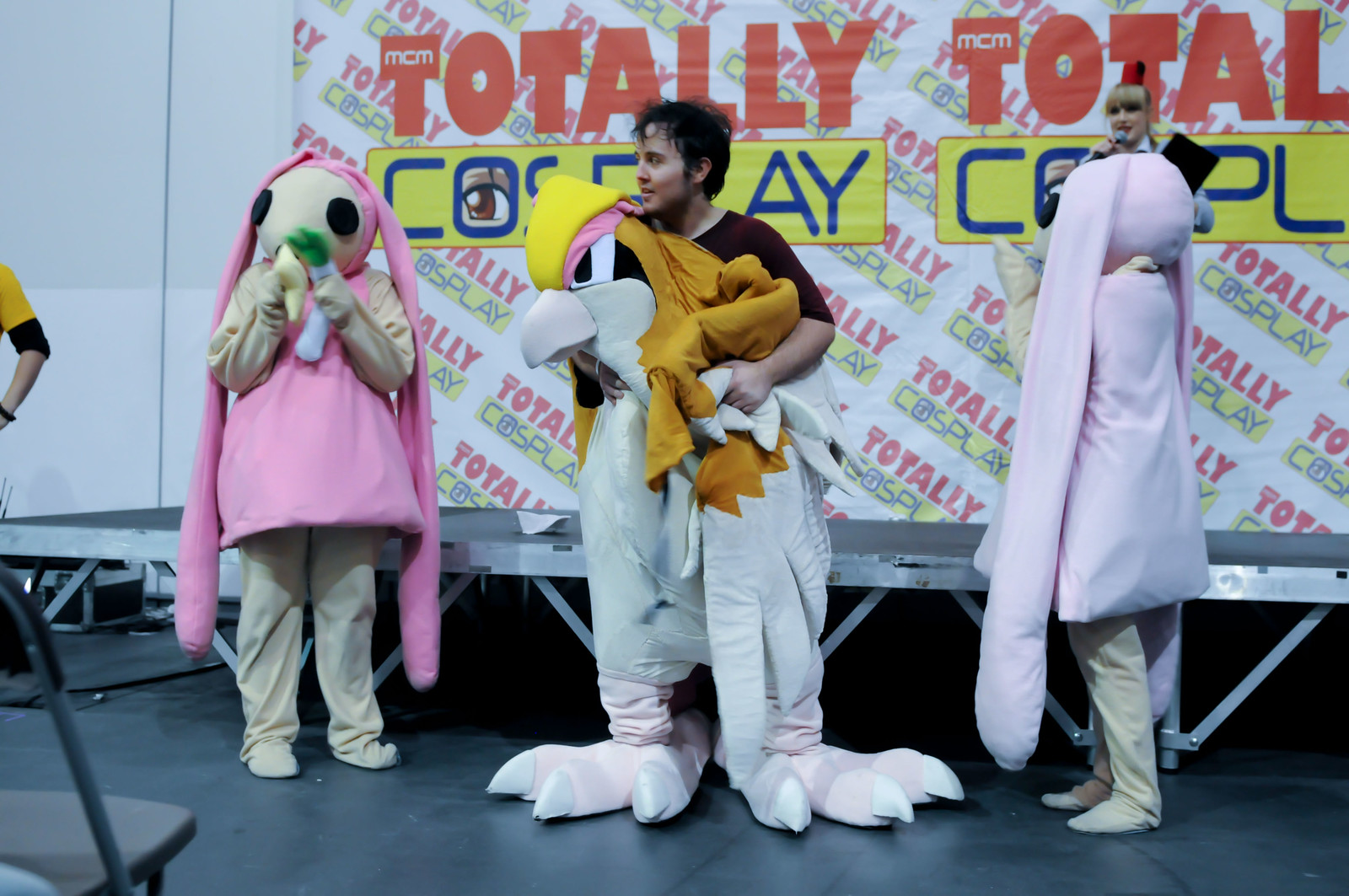In this detailed photograph, three individuals are positioned in front of a stage at a cosplay exposition, as indicated by a "Totally Cosplay" banner in the background with the word "Totally" in red and "Cosplay" in blue and yellow. Flanking the scene are two people dressed in bunny costumes; the bunny on the left is medium pink with very long ears that stretch from the top of their head almost down to their ankles, paired with tan pants. The person on the right is also dressed as a bunny but in a slightly different shade of light pink with enormous black eyes and similarly lengthy ears. 

Centrally positioned is a gentleman who appears to be in the process of removing a costume. He sports large clawed pink feet and gray bottom legs, indicative of a bird-like outfit. He holds a bird's head piece in his hand, and his disheveled hair suggests he has just taken it off.

On the stage, partially obscured by one of the bunny costumes, is a person holding a microphone, engaged in speaking. The scene captures the lively and whimsical atmosphere of the cosplay event.